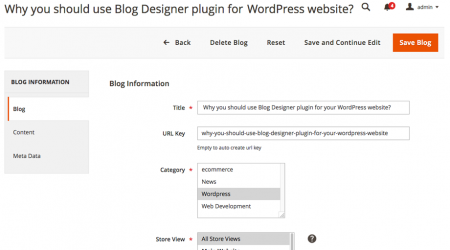The image features a clean white background with prominently displayed black text at the top reading, "Why You Should Use Blog Designer Plugin for Your WordPress Website." Below this heading, there are three icons: a magnifying glass, a bell with one alert, and a sign-in button. 

Directly underneath these icons, a set of black tabs are listed: "Back," "Delete Blog," "Reset," "Save and Continue Edit." On the right side, an eye-catching orange button labeled "Save Blog" stands out. 

Beneath this, the background continues to be white. On the left, there is a light grey column with black text reading "Blog Information." Under this heading, there are two selectable options: "Blog" and "Metadata," with "Blog" currently selected.

In the center of the image, also against a white background, the text "Blog Information" is once again in black. Below this heading, there are several labeled input boxes. The first box, titled "Title," contains the text "Why You Should Use Blog Designer Plugin for Your WordPress Website." Next is the "URL Key" box which provides the URL. The "Category" section follows, listing several options: "e-commerce," "news," "WordPress" (which is selected), and "web development." Lastly, the "Store View" section includes the option "All Store Views," with this option currently selected.